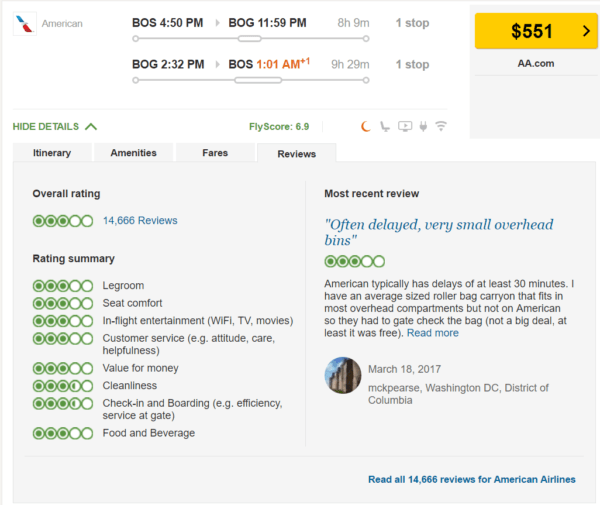This image predominantly square in form, is slightly wider than it is tall, and features a light gray border outlining its perimeter. The image showcases a screenshot of a travel website or application, likely dedicated to booking airfare, specifically highlighted by the American Airlines logo and the word "American" in small, gray font in the upper left corner.

The main content of the image details a planned trip. The itinerary starts with a departure from Boston at 4:50 PM, followed by a gray arrow indicating the next destination as BOG, which corresponds to El Dorado International Airport in Bogota, arriving at 11:59 PM. This segment of the trip totals eight hours and nine minutes with one stop. Below this information, the return flight is displayed: departing from BOG at 2:32 PM and arriving back in Boston at 1:01 AM the following day, denoted by a "+1" in orange next to the arrival time. This return trip is nine hours and twenty-nine minutes long, also featuring one stop.

Additionally, the lower section of the image presents navigation options such as "Itinerary," "Amenities," "Fares," and "Reviews," accompanied by ratings for various aspects of the flight experience.